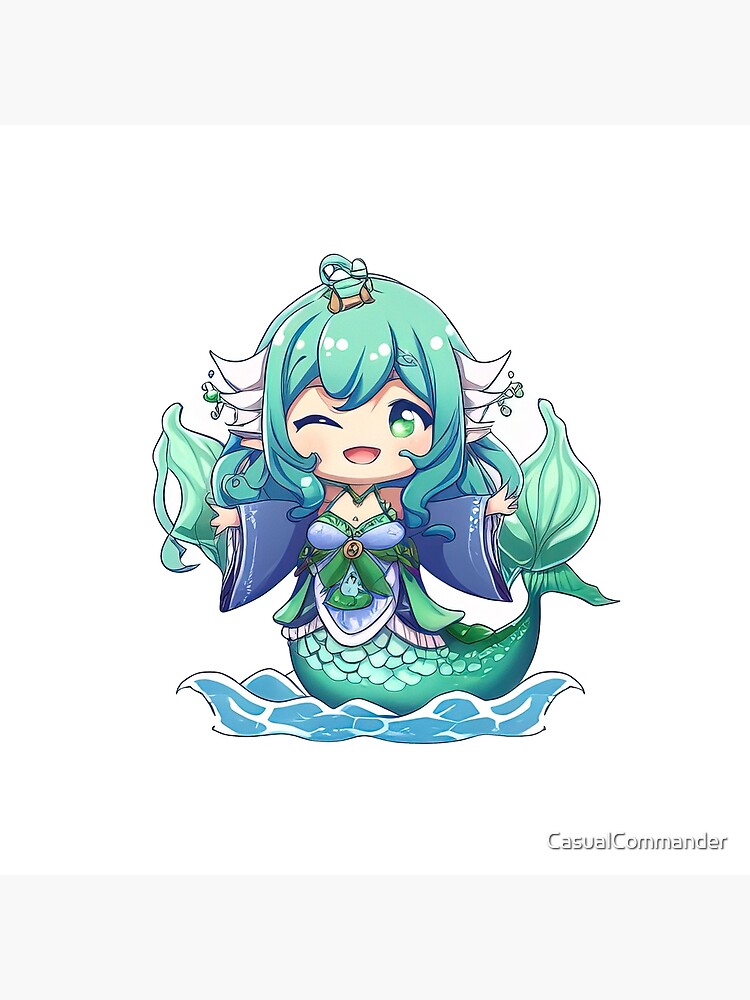This illustration depicts a mermaid in Japanese anime style, floating on a body of blue water with white caps, detailed with ripples and waves. She has long, teal blue hair accented with dark teal and white highlights. Adorning her hair, she sports a ribbon, and three ornamental curls extend from the sides of her head. Her face features one closed left eye and an open right eye, both in green, with her mouth open and no visible nose.

Dressed in a blue kimono with light blue and green accents, she wears a loose-fitting coverall across her chest. There is a bow between her breasts, embellished with a small metal medallion, suggesting an open kimono with a spaghetti strap top beneath. Her body is covered in scales, and her turquoise tail, shaded in teal, curves upward, akin to a boat shape. The character extends her arms outward, as if in motion or speaking. Surrounding her are flowing light green waves or seaweed-like elements.

The image includes a notation in the lower right-hand corner that reads "Casual Commander" in capitalized white letters with a shadow effect, enhancing its visibility against the predominantly blue and white background.